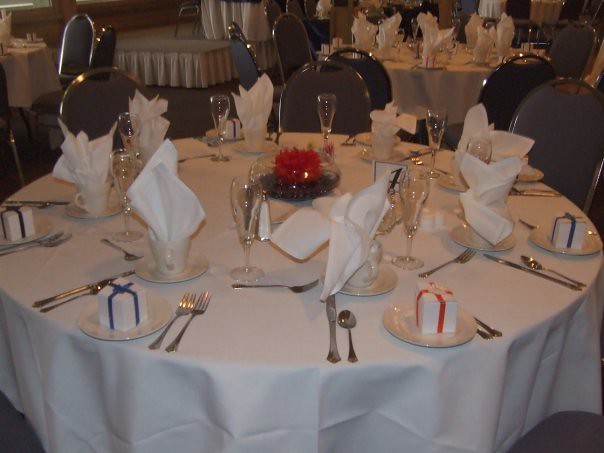In this dimly lit photograph, we see a large, round table set up in what appears to be an event hall, possibly for a wedding or similar celebration. The table is draped in a pristine white tablecloth, with ten elegant place settings evenly spaced around it. Each setting includes a white plate accompanied by neatly arranged silverware, a coffee mug with a fanned-out napkin, and a wine glass. At the center of each plate sits a small, white gift box adorned with a ribbon, mostly red though one description mentioned blue as well. The table is further adorned with a centerpiece featuring a glass bowl filled with vibrant red flowers. Surrounding this main table are at least three identical tables, each with black chairs positioned for the guests. A white card marked with the number one indicates this might be the main or designated table. The overall ambiance suggested by the setup indicates an upcoming festive gathering.